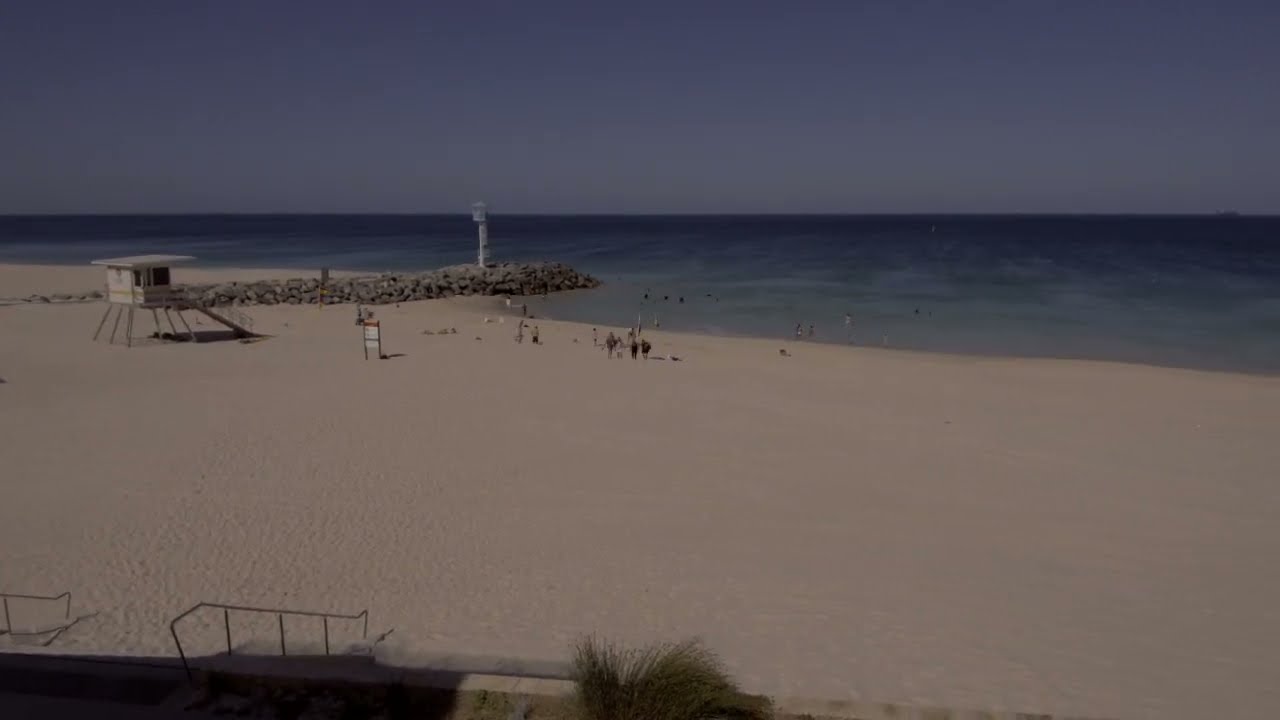This color photograph, captured from a higher vantage point possibly on a second or third-story beachfront hotel balcony, showcases a serene and expansive beach scene. The image, although somewhat blurry and not of high quality, highlights a vast, clean expanse of pinkish-beige sand, occupying the bottom 70% of the frame. This smooth and mostly untouched sandy area is dotted with a handful of beachgoers walking near a small rock jetty that extends about 20 feet into the ocean. On the center left of the image stands a white lifeguard tower, resembling a small, elevated hut accessible by stairs, poised to monitor the calm, clear waters. The ocean, a soothing blue, extends into the pale blue sky, creating a tranquil and picturesque backdrop. At the bottom left, a hint of a railing and some grass indicates the walkways leading towards this idyllic beach. Overall, this photograph effectively captures a beautiful day at the beach, with people enjoying the tranquil environment, punctuated by a subtle presence of signs and the functional architecture of the lifeguard tower.